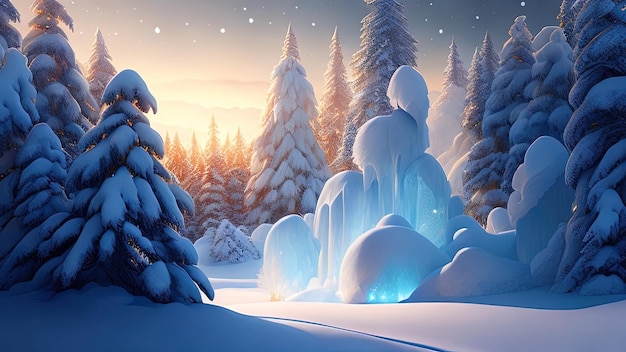The digital illustration depicts a serene winter landscape featuring a dense forest of snow-covered coniferous trees. At the center of the image stands a structure that resembles a snow fort or castle, characterized by its domed roofs and a mysterious, glowing blue light emanating from within. A blanket of white snow covers the ground, creating a contrast with patches of brighter turquoise hues in certain areas. The sky, painted in shades of gray and light blue, is dotted with white stars or falling snowflakes. The setting sun casts a golden light from the left side of the scene, illuminating the snowy path that winds through the trees and casting an ethereal glow over the entire illustration.